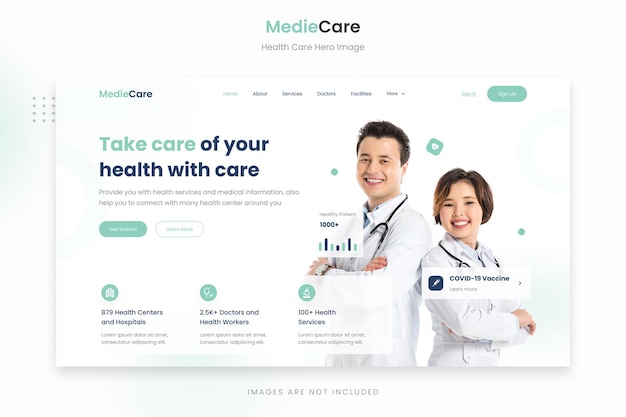The image features a sleek, modern homepage design for a healthcare service platform named "Medi-A Care." The brand logo, "Medi-A Care," is displayed prominently, with "Medi-A" in a light green color and "Care" in dark blue. Below the logo, a tagline in gray reads "Health Care Hero Image."

The webpage layout is organized, with a navigation menu at the top listing options: "Home," "About," "Services," "Doctors," "Facilities," and "More." On the right side of the menu, there are buttons for user actions, including a "Sign In" link and a green "Sign Up" button.

A bold, large headline in the center of the page proclaims, "Take Care of Your Health with Care." Below this, a gray subtitle explains the platform's offerings, stating: "Provide you with health services and medical information. Help you to connect with many health centers around you." 

A prominent green "Get Started" button and a "Learn More" button in white are positioned side by side underneath the text.

The page highlights three key statistics: 
1. "879 Health Centers and Hospitals" with descriptive text below.
2. "2.5K+ Doctors and Health Workers" accompanied by additional information.
3. "100+ Health Services," each category depicted with a small green icon above it.

To the right side of the page, an image showcases a male and a female doctor, both dressed in white coats with stethoscopes around their necks. They are smiling confidently with their arms crossed. Above the male doctor, an icon indicating "COVID-19 Vaccine" is displayed.

At the bottom of the image, a note clarifies: "Images are not included."

Overall, the caption comprehensively describes the visually appealing and informative layout of the "Medi-A Care" healthcare platform's homepage, emphasizing its features and user-friendly interface.